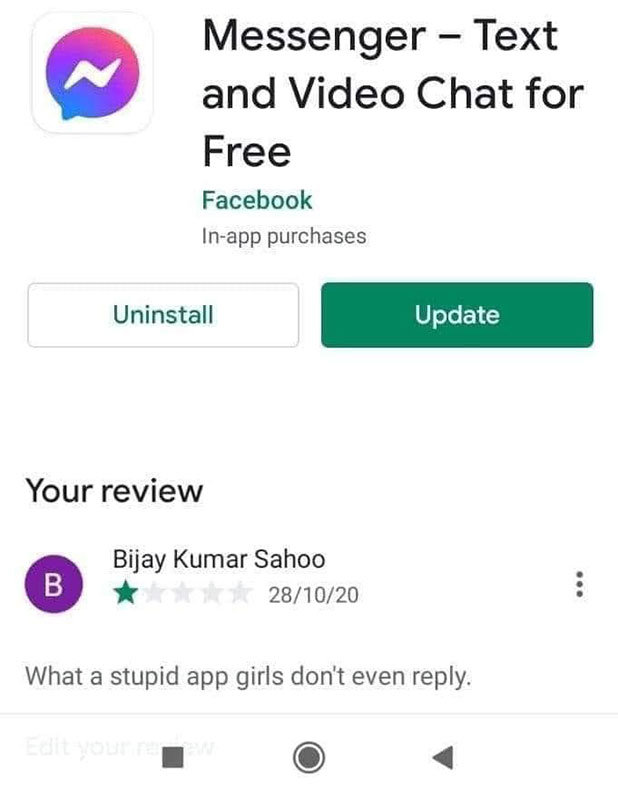**Screenshot Description: App Library**

The image is a detailed screenshot taken from an app library on a mobile device. At the center of the screenshot, there is the app "Messenger - Text and Video Chat for Free," which is identified as a Facebook product. The description beneath the app indicates it includes in-app purchases.

To the right of the app description, there's a prominently displayed green button labeled "Update," suggesting that an updated version of the app is available for download. On the left side, there is a white button labeled "Uninstall," giving the user an option to remove the app from their device.

Below the update and uninstall options, there's a section labeled "More review." In this review section, a user's feedback is shown. The review is by "Vijay Kumar Sahu," who rated the app one star on October 28th, 2020. Vijay's critical review reads, "What a stupid app, girls don't even reply."

This snapshot provides a clear view of the app's details, update status, and user feedback, highlighting both functionality and user sentiment.